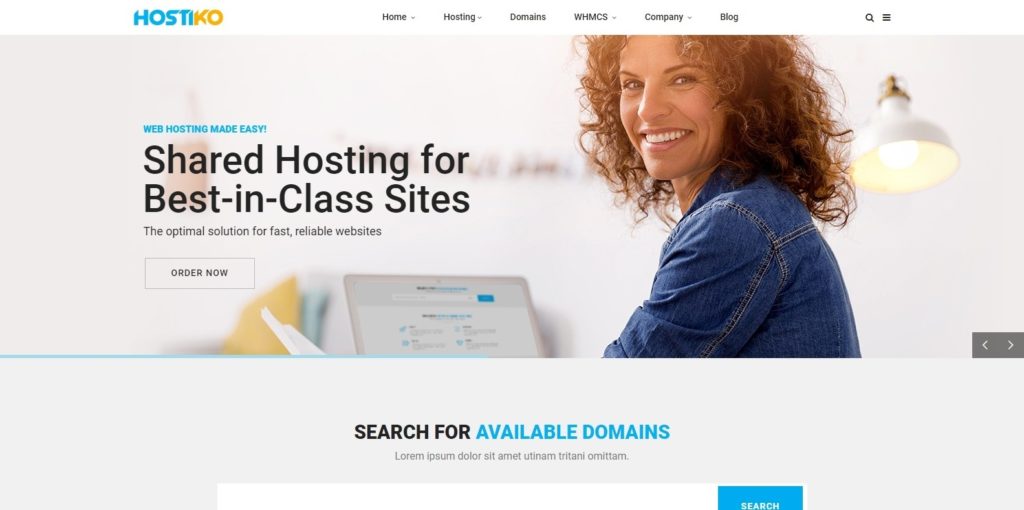The image features a website interface for Hostiko, a web hosting service. The prominent Hostiko logo is displayed at the top left, with 'Host' in blue and 'iko' in orange. The main visual element is a woman sitting at a laptop; she is turned around, smiling brightly at the camera, showcasing her white teeth. She is dressed in a denim jacket. 

To the left of this central image, small text reads "Web hosting made easy!" exclaiming the simplicity of their service. Below this, in large black text, it states "Shared Hosting for Best in Class Sites." Further down, it elaborates with "The optimal solution for fast, reliable websites," accompanied by an 'Order Now' button.

Centered below this text, there is a search bar instructing users to "Search for available domains" in blue and black text, followed by a different language translation. The search bar partially reveals a search icon, indicating a truncated view. At the bottom right corner, arrows suggest additional images of Hostiko can be viewed.

Additionally, the top section of the webpage, positioned to the right of the Hostiko logo, includes navigation options such as "Home" with a dropdown menu, "Web Hosting," "Domains," "WHMCS" (possibly referring to web hosting management software), "Company," and "Blog Information." A search icon is situated at the far right, next to a three-horizontal-line menu icon for settings.

In the background of the image, there is a wall-mounted lamp and a shelf or table with books, adding a cozy, productive atmosphere to the scene.